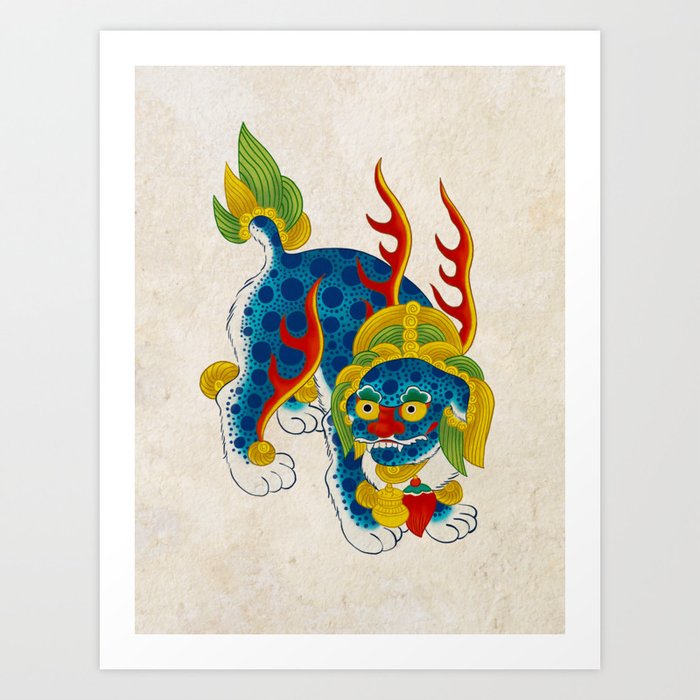The image depicts a vibrant painting set against a cream-colored background with a white outline and a light gray border. At the center is an intriguing creature, a blend of dog and dragon attributes, standing on all fours, its gaze slightly off to the right. The creature's body is primarily light blue with dark blue leopard-like spots, and its white paws contrast starkly against its colorful fur.

The face features striking yellow eyes with black pupils and bushy green eyebrows, enhancing its fantastical appearance. A red human-like nose and a white mouth with jagged teeth add to its uniqueness. Surrounding its head is a golden and green mane, reminiscent of flowing spaghetti, contributing to the creature’s majestic demeanor.

Flaming orange and yellow horns sprout from its head, while red and orange wing-like flames emerge near its shoulder blades and back paws, adding a dynamic, mythical element to the creature. The short tail flares outward, adorned with yellow and green leaf-like symbols, completing the fantastical portrayal of this dog-dragon hybrid.